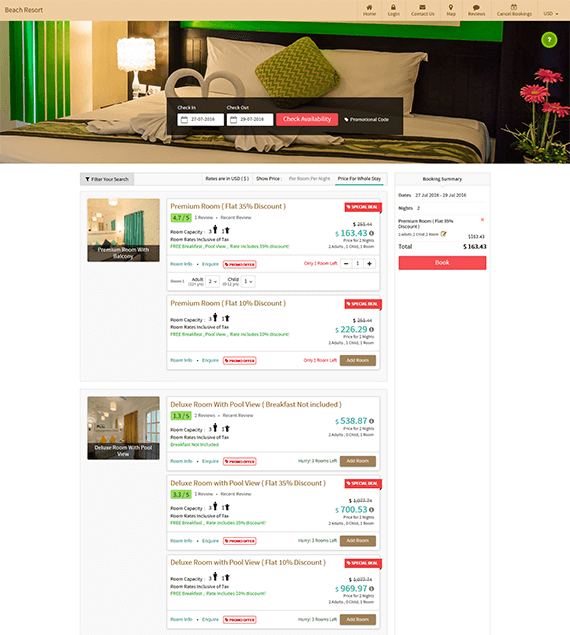The screenshot showcases a detailed composition of a webpage interface. At the top, there is a light brown rectangular header adorned with light black icons on the right, each with a corresponding label. Beneath the header is a photograph of a neatly made bed. The bed boasts a black headboard and is adorned with two white pillows flanking a central green square pillow. The bedspread and sheets feature a blanket with a green border at the top edge. On the right side of the bed, three vibrant red-pink daisies provide a pop of color. To the left, a lit lamp sits on an unseen nightstand, casting a warm glow. Adjacent to the lamp, a beige wall with green curtains is visible.

Below the photograph, the screen displays a menu resembling search results. This section includes two gray rectangles stacked vertically. Each rectangle features an image of a room in the upper left-hand corner, accompanied by a white rectangle filled with room information. At the top right, a gray square with black text is visible, followed by a prominent red rectangle stretching across the bottom of the section. This detailed arrangement provides a clear visual and informational hierarchy.